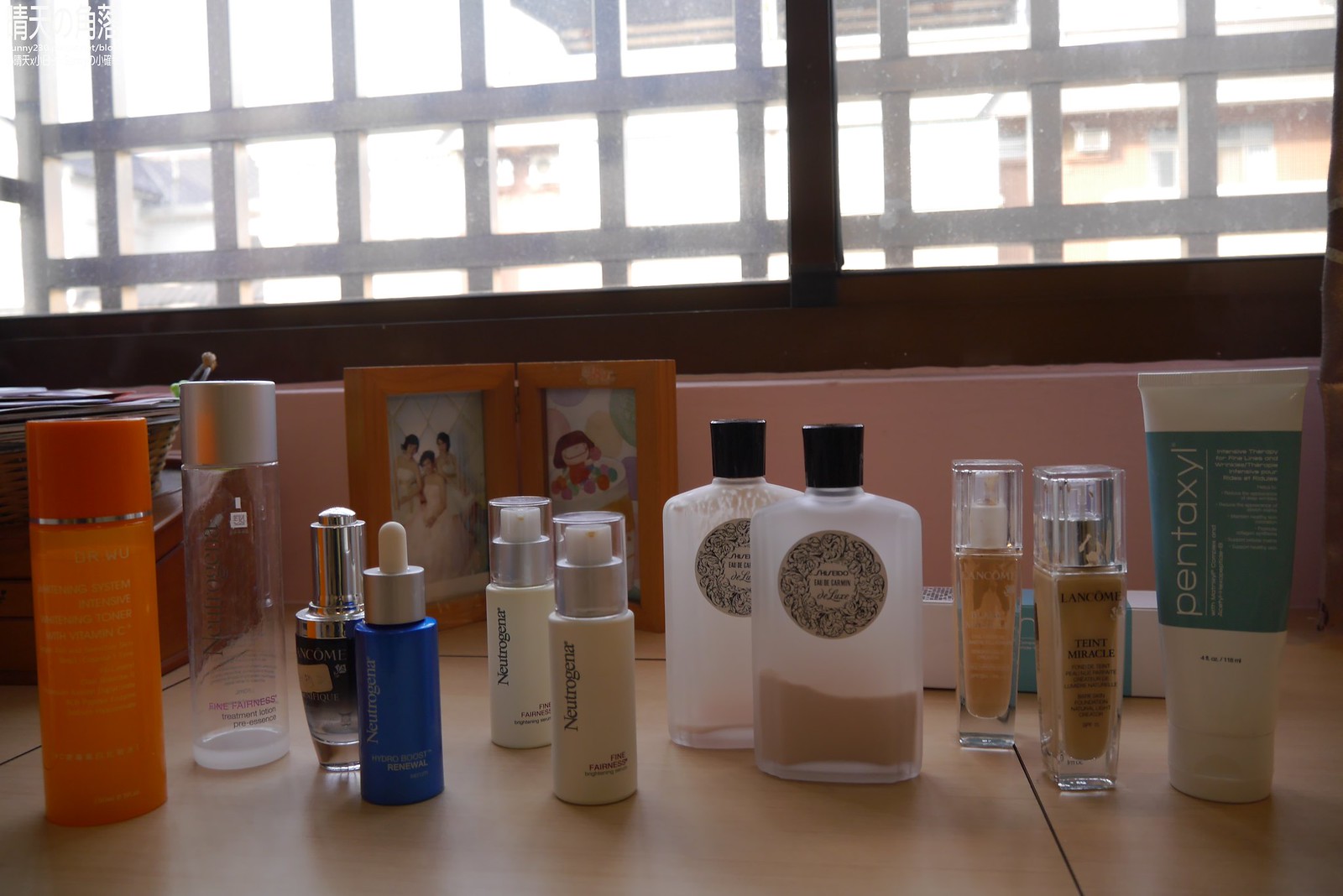This image depicts an organized makeup table situated beneath a window with distinctive wooden crisscross designs. The table features an array of cosmetic and skincare products, including various lotions, facial and body care items, foundations, and primers. Among the recognizable brands, Neutrogena products are prominently displayed. Additionally, there is a prominent orange bottle, possibly Kleenex perfume. The table also includes some personal touches, such as a double picture frame showcasing artistic drawings and a box of Kleenex tissues. Some products appear in both new and used conditions, indicating regular use. The natural light from the window enhances the visibility and overall ambiance of the makeup setup.